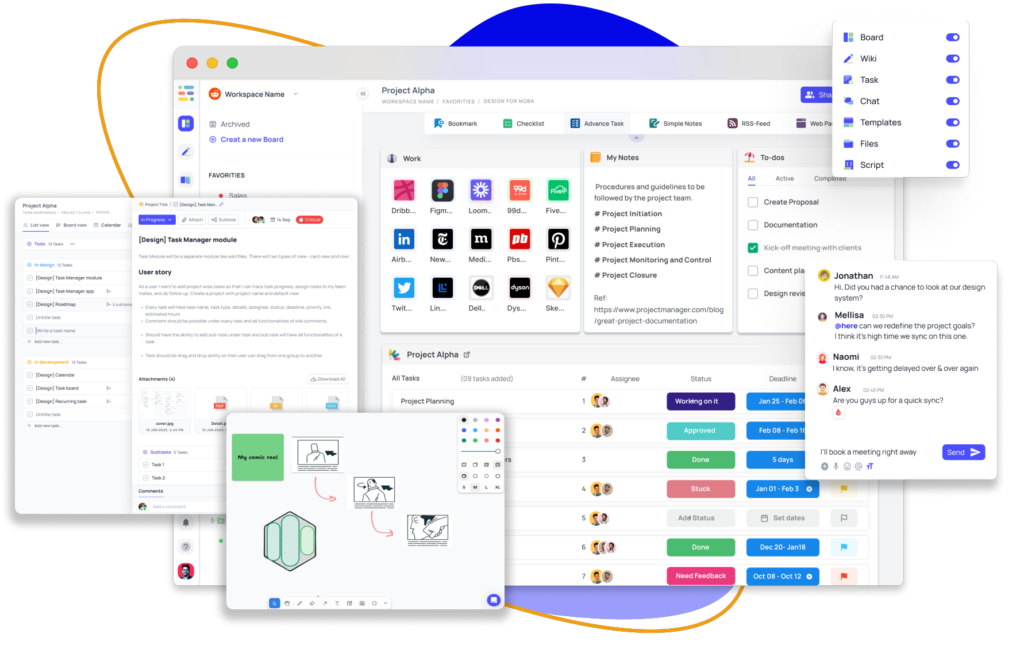The image depicts a computer screen with multiple browser tabs, with the primary focus on a main tab titled "Project Alpha." This main tab is well-organized and segmented into various sections and functionalities. 

At the top of the main tab, there's a section labeled "Work," which features a series of symbols representing different websites. Adjacent to it is a "My Notes" tab, followed by a "To Do" section. Below these sections, the title "Project Alpha" appears again, listing various tasks, although the specific tasks are illegible due to the small print.

In the upper right corner of the screen, a small elevated box displays several toggles for different features. These include "Board," "Wiki," "Took," "Chat," "Templates," "Files," and "Script," all of which are activated.

Another box on the screen reveals a conversation among several users. Jonathan initiates the dialogue with, "Hi, do you have a chance to look at our design system?" Melissa responds, though her complete reply is unreadable. Naomi follows with a comment about the ongoing delays, and Alex asks if the team is available for a quick synchronization. The owner of the screen is in the process of typing the message, "I'll book a meeting right away," but hasn't sent it yet. A send button is present to dispatch this message to the group chat.

On the left-hand side of the screen, two additional tabs are open, though the text is too small to discern their contents.